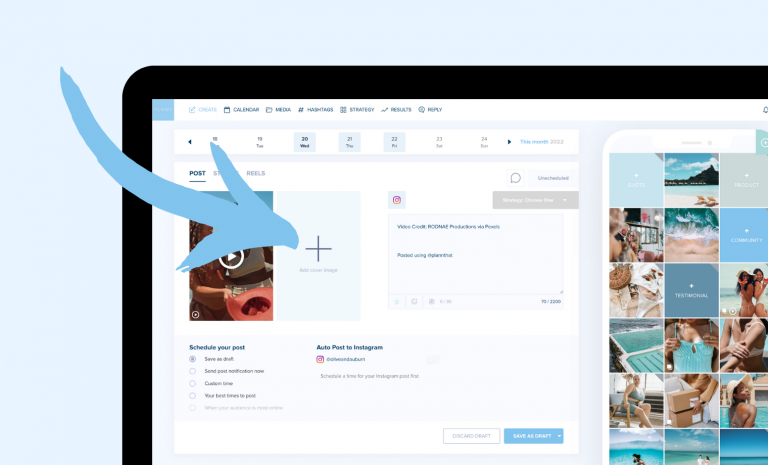In this detailed image, captured from a digital device, there's a distinctive graphical overlay. A blue arrow starts from the upper left-hand corner, curving down and around to point directly at a bold plus sign located in the center-left area of the screen. The upper portion of the image is filled with a light blue color, which extends down the left side, providing a calming backdrop.

The device's interface features a thin, black rectangular outline on the top and left edges, framing the content within. Adjacent to the plus sign, a video is visibly playing, adding dynamic visual interest.

On the right-hand side, a cell phone is displayed prominently, showcasing a variety of images. These images include vibrant beach scenes, individuals relaxing on chairs, a person donning a stylish sun hat, and several idyllic vacation photos with water elements. These pictures occupy the lower right corner, creating a collage of serene, sun-soaked memories.